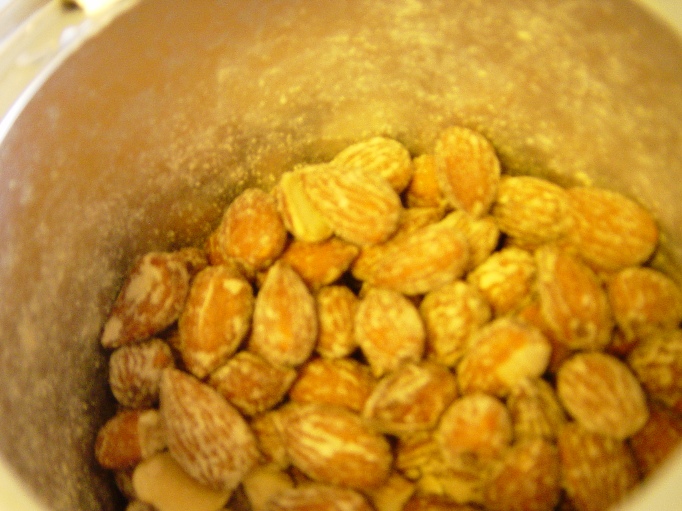This close-up photograph features a round container, likely made of clay or terracotta, with a somewhat worn, beige interior. Inside the container are approximately a cup to a cup and a half of nuts, which appear to be roasted. While there is some ambiguity around the type of nuts, they might be small almonds, peanuts, or another similar variety. The nuts have a light brown, dried appearance characteristic of being roasted. They are coated or seasoned with some type of yellow powder, possibly butter seasoning, giving them a slightly yellowish tint. The coating also contributes to the dusting on the inner walls of the container, suggesting that the nuts are well-seasoned and ready to eat.